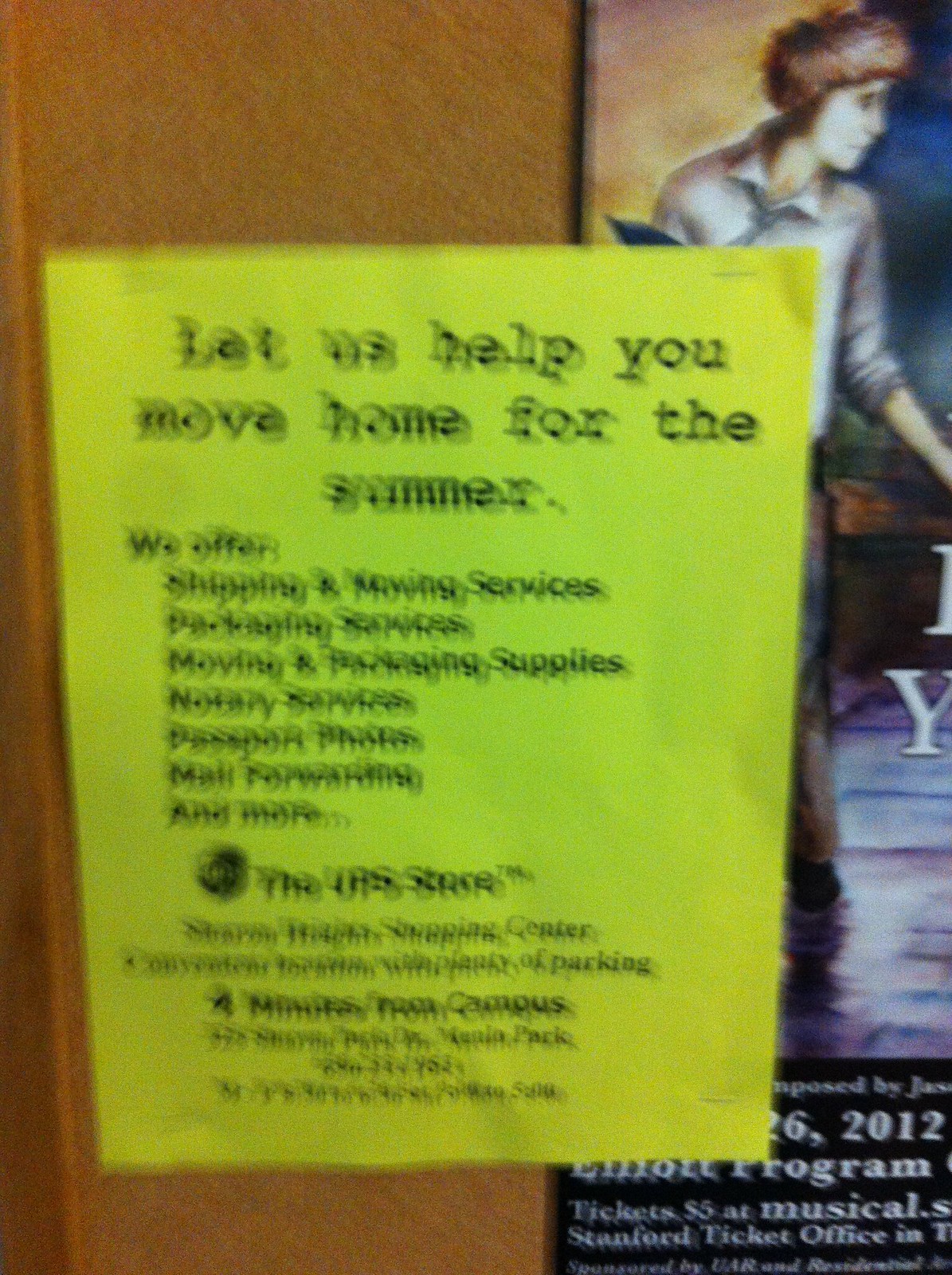The image is a blurry snapshot taken in what appears to be a hallway at Stanford University, possibly in a dorm or academic building. The photo captures a cork bulletin board framed in wood, visible on the left side. Mounted on the board is a poster, partially obscured by a neon yellow flyer. The poster, situated on the right side of the image, advertises a Stanford program with tickets priced at $5, featuring a young man with brown hair in an unbuttoned white collared shirt. The date "2012" and the term "Elliott Programs" are partially legible, suggesting a musical event.

Overlapping this poster, a bright yellow flyer from The UPS Store prominently advertises summer moving services. The text reads: “Let us help you move home for the summer. We offer shipping and moving services, packaging services, moving and packing supplies, notary services, passport photos, mail forwarding, and more.” Below this, additional blurry text provides more details likely about store locations or further contact information. The entire image, including both the poster and the flyer, is marked by poor focus, making the finer details difficult to discern.